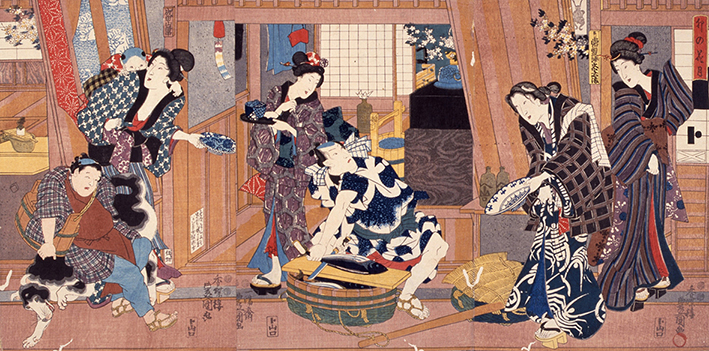This vibrant Japanese-style watercolor painting depicts a busy scene in a traditional Japanese house filled with activity and intricate details. There are six women, each adorned in richly textured, colorful garments featuring patterns such as flannel, stripes, and spots. 

On the left, one woman stands with a baby on her back while another crouches beside her, placing a hand on a dog. The central pair consists of a woman standing and holding a fish, with another woman leaning backward over a tub, seemingly busy with laundry. The rightmost pair shows two women standing; one is nearly dropping a blue and white porcelain bowl, while the other clutches an object, possibly a pillow, close to her body.

The background reveals multiple rooms of the house, including a dining room with windows and a hallway, adding depth to the scene. The overall atmosphere is one of chaotic commotion as the women navigate clumsy clutter and various household tasks, vividly capturing a moment of everyday life brimming with activity and detail.